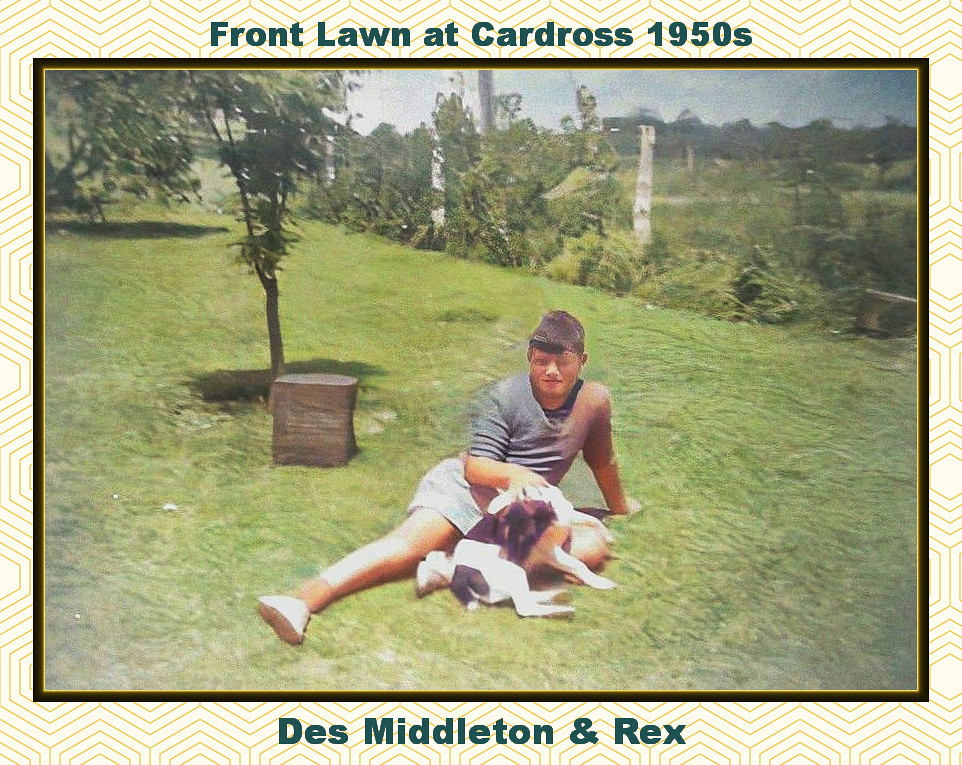This photograph, titled "Front Lawn at Cardross, 1950s," captures an idyllic outdoor scene punctuated by its distinctiveness and nostalgic charm. It is presented within a rectangular frame, bordered by a pinstripe yellow line and a slightly thicker black line, followed by a light tan border adorned with a pattern of repeating yellow hexagons. The image itself displays a slightly slanting grass-covered hill that descends from the upper left to the lower right.

At the center of the photograph, a boy approximately 12 to 14 years old of Caucasian descent lays on the grass. He has short brown hair and is dressed in a short-sleeved t-shirt paired with light-colored shorts. Despite the aged and slightly distorted quality of the photo, it clearly shows the boy with his hand affectionately resting on a black and white dog that is curled up beside him. 

To the left of the boy and dog lies a brown tree stump or possibly a can, with a small sapling growing behind it. In the upper right corner of the photograph, the blue sky stretches above a distant city skyline visible beyond the hill. Additionally, a wire fence intertwined with bushes can be discerned in the background. The header in green print reads "Front Lawn at Cardross, 1950s," while the footer centrally displays the names "Des Middleton and Rex."